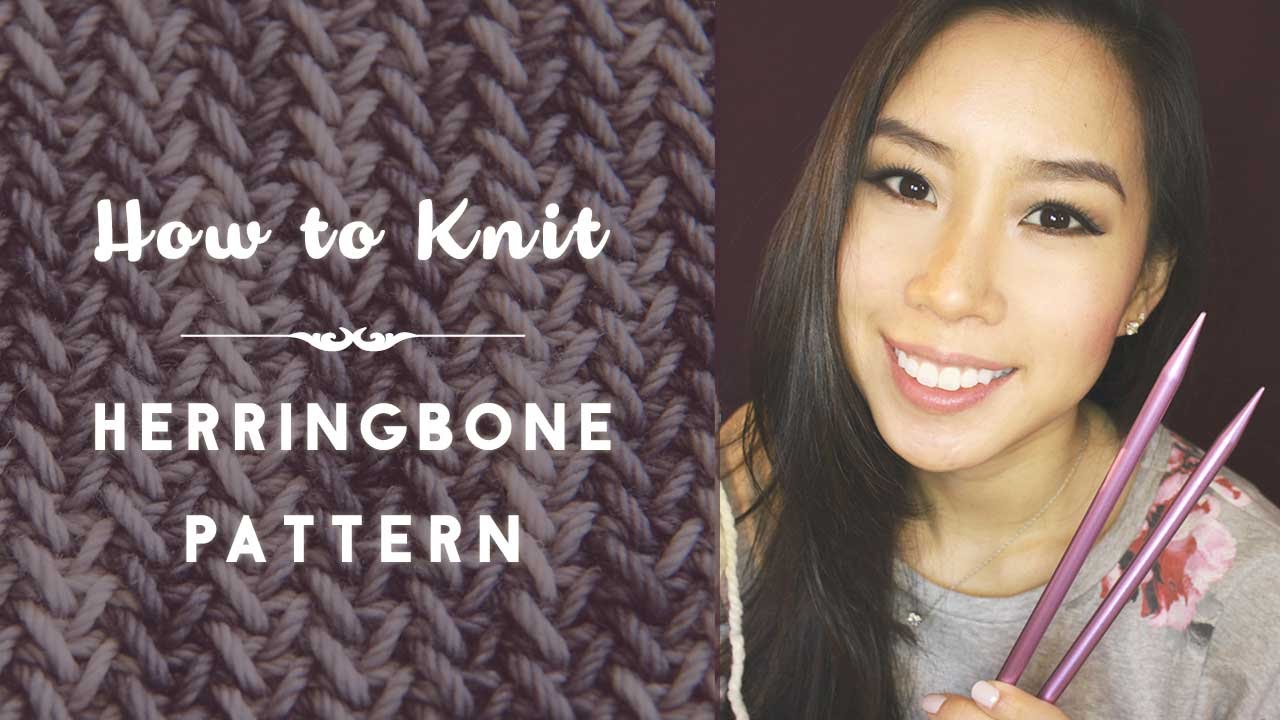This detailed photograph resembles a poster or tutorial advertisement. It features a close-up of an Asian woman with long, straight black hair, smiling widely to reveal her white teeth. She is positioned on the right side of the image and is holding two pinkish-purple knitting needles in her left hand. She wears a gray shirt adorned with large pink flowers. The background behind her is black, allowing her figure to stand out prominently.

On the left side of the image is a close-up of a knitted fabric in a plum-colored herringbone pattern. Superimposed on this fabric is the text "How to Knit HERRINGBONE PATTERN." The phrase "How to Knit" is written in cursive, while "HERRINGBONE PATTERN" is in bold, capital letters. All the text appears in white, providing a striking contrast against the darker, plum-colored knitwear. This comprehensive display makes it clear that the woman is promoting a tutorial or method for knitting the herringbone pattern.